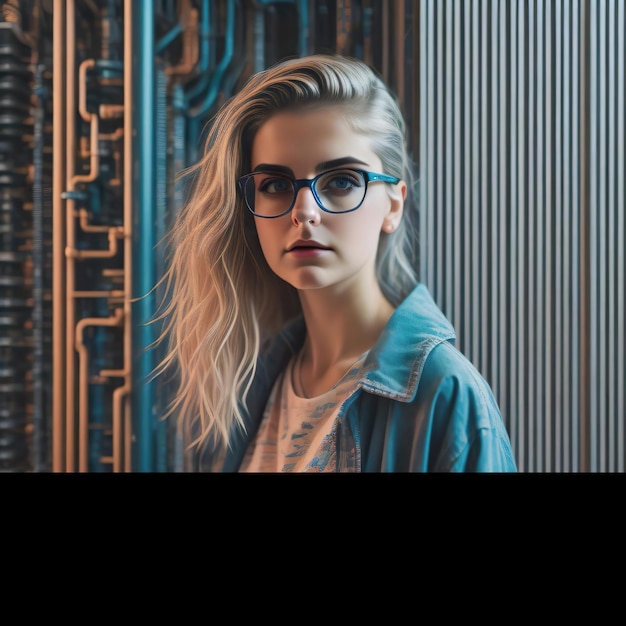The image features a detailed portrait of a young blonde woman looking directly at the camera, possibly a highly realistic AI-generated painting. She is wearing stylish blue-rimmed glasses and a denim jacket over a predominantly white top with subtle black accents. Around her neck, she seems to have a strand of pearls. Her hair is swept to her right, exposing her left ear and cascading slightly below her shoulders. The backdrop presents an artistic and industrial vibe, with a series of vertical pipes in shades of pink, blue, and silver set against a black background to the left. On the right, a wall with vertical blue and black stripes and a coiled structure further enhances the modern aesthetic. The bottom section of the image includes a solid black band, possibly serving as a placeholder. The overall composition emphasizes the eyewear she is modeling, underlined by her direct gaze and the intricate background elements.